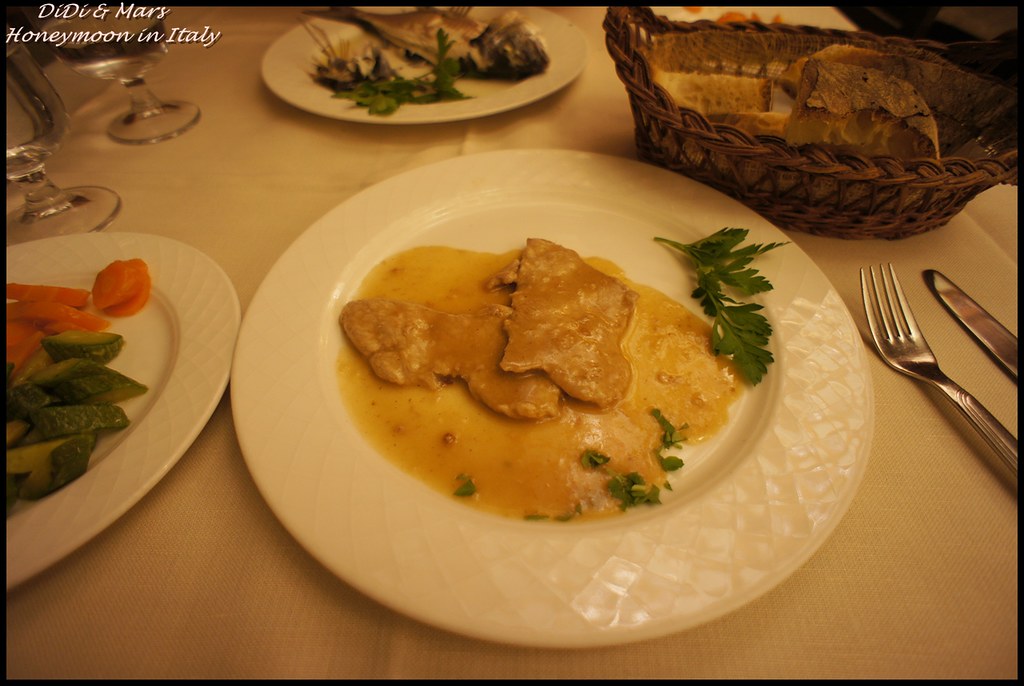This indoor photograph, framed with a thin black border and labeled "D.D. and Mars Honeymoon in Italy" in white print in the top left corner, showcases a rectangular table setting viewed from above. The central focus is a large white plate with slightly textured, diamond-patterned edges. The plate presents 'scallopini,' featuring thin slices of meat draped in a light brown sauce, garnished with green cilantro leaves. To the left, partially off-screen, sits a slightly smaller white plate adorned with neatly sliced carrots and zucchini. On the right side of the photo, a silver fork and knife are positioned at an angle, partially extending out of the frame. In the upper right, a small brown basket filled with thick, slightly hard bread is visible. Centered at the back of the table, another white plate holds a whole fish, complete with the head and garnished with parsley. Lastly, beneath the text in the upper left, two glass cups of water can be seen.